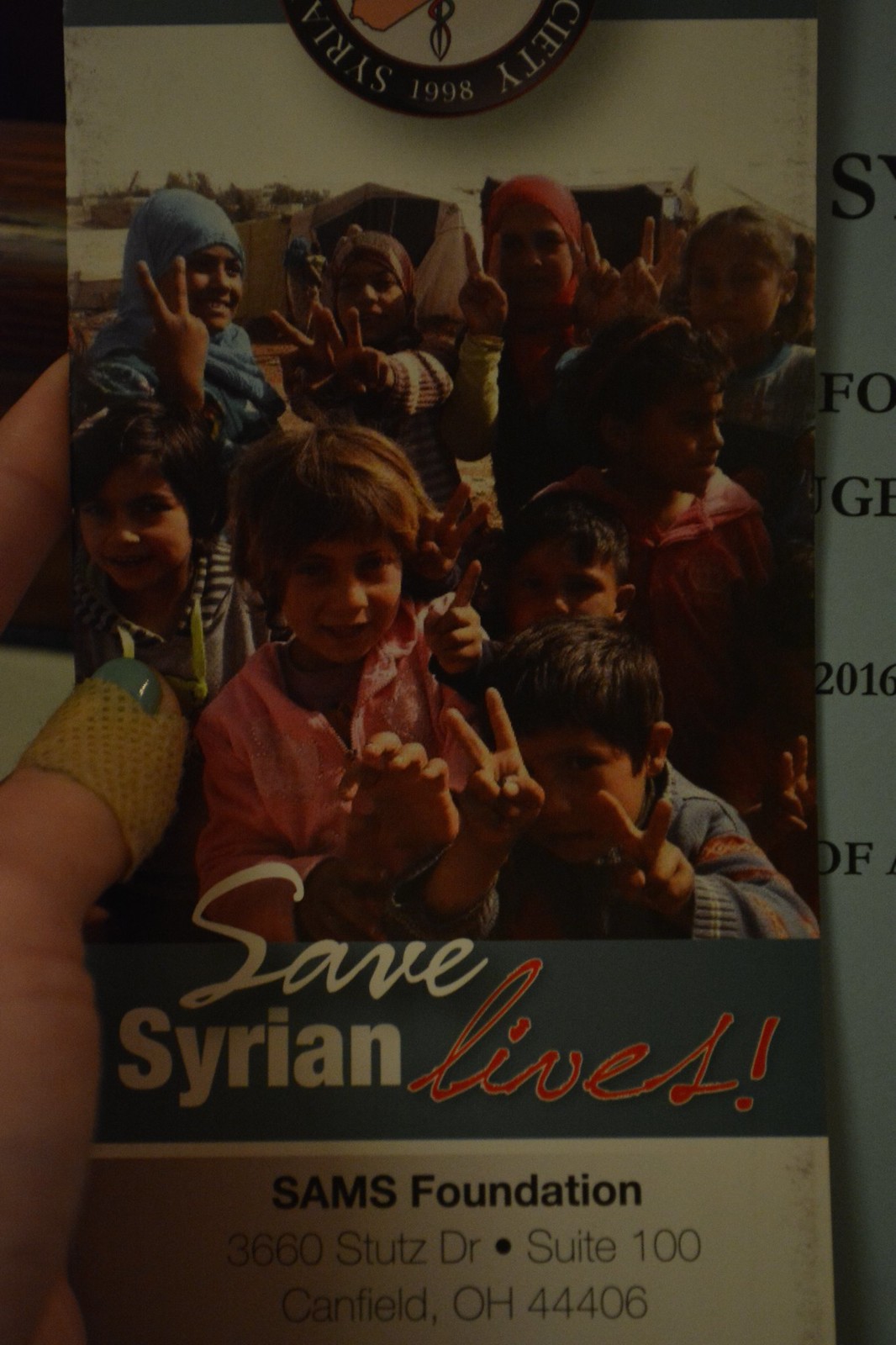In the photo, a close-up shot reveals a person holding a brochure in their left hand. The person has a band-aid on their thumb, which is covered in blue-pinkish nail polish. The brochure prominently displays a group of smiling children, approximately nine or ten in number, many of whom are making peace sign gestures toward the camera. Behind the kids, there is a faint image of what seems to be tents, suggesting a refugee setting. The top of the brochure reads "Syrian and society, 1988" with the text partially cut off, and at the bottom, the words "Save Syrian Lives" stand out, with 'Lives' in red and 'Save Syrian' in white. Also visible is the address "SAMS Foundation, 3660 Stutz Drive, Suite 100, Canfield, Ohio, 44406." In the background, a separate paper with letters possibly relating to Syria is partly visible.